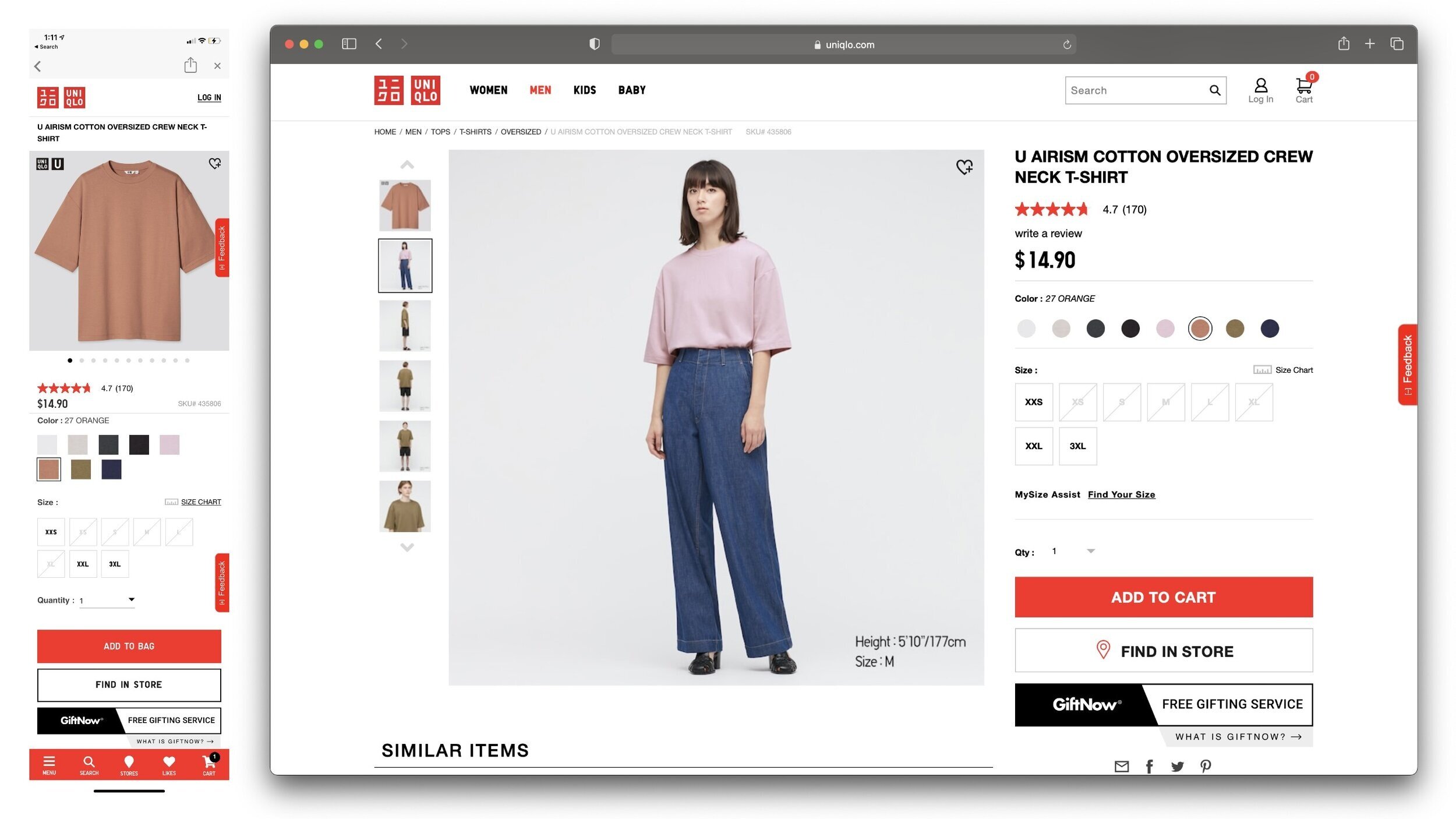This image showcases a fashion website, presented in both mobile and desktop views. 

In the mobile view, located at the top left, there is a distinct gray banner with a gray arrow, which likely includes information such as the current time, although it is not clear. Icons for uploading and exiting are visible on the right-hand side of this banner. Below this, on the left, there are two boxes with unreadable symbols, and to the right, a "Log In" button. Beneath these elements, a descriptive sentence appears, followed by an image of a brown shirt, priced at $14.99. This section also includes product ratings, color options with the brown shade selected, size selections, and two action buttons: a red "Add to Bag" button and a white "Find in Store" button. The brand name, possibly "GNU," is displayed in black text. At the bottom, there are several icons.

The right half of the image depicts the desktop version of the same fashion website. The page header features categories like "Women," "Men" (currently highlighted), "Kids," and "Baby." Below, there is an image of a woman wearing blue pants and a pink elbow-length sleeve shirt. On the left section of the screen, there are different images showing various angles of this shirt. The product description on the right reads "Cotton Oversized Crewneck T-Shirt," priced at $14.90, and matches the information provided in the mobile view section.

Overall, the image captures a detailed view of an e-commerce fashion webpage, highlighting key features such as product images, pricing, size and color options, and navigational elements for both mobile and desktop interfaces.